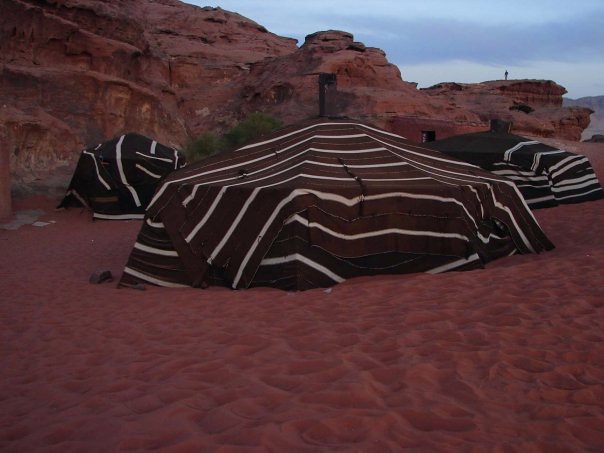The photograph showcases a striking outdoor scene in a desert environment with vibrant red clay sand scattered across the ground. Three octagonal tents, all designed with contrasting brown or black fabric accented by white stripes, stand prominently in the red sandy area. One tent appears to have a chimney emerging from its center, adding a unique feature to the campsite. The perspective of the image suggests it was taken during the late day, nearing dusk, as the sky above is a light blue interspersed with dark gray clouds, signaling the waning daylight. 

In the background, towering rocky cliffs with multiple layers and large boulders create an imposing natural backdrop. In the top right corner of the image, a person can be seen standing on one of the cliffs, gazing outward, adding a sense of scale to the vast landscape. The red sand in the foreground shows visible signs of previous foot traffic, indicating human activity in the area. Additionally, at the edge of a rock wall, there appears to be a doorway carved into the cliff, suggesting a makeshift room built into the rock face, hinting at more permanent human presence in this rugged setting.